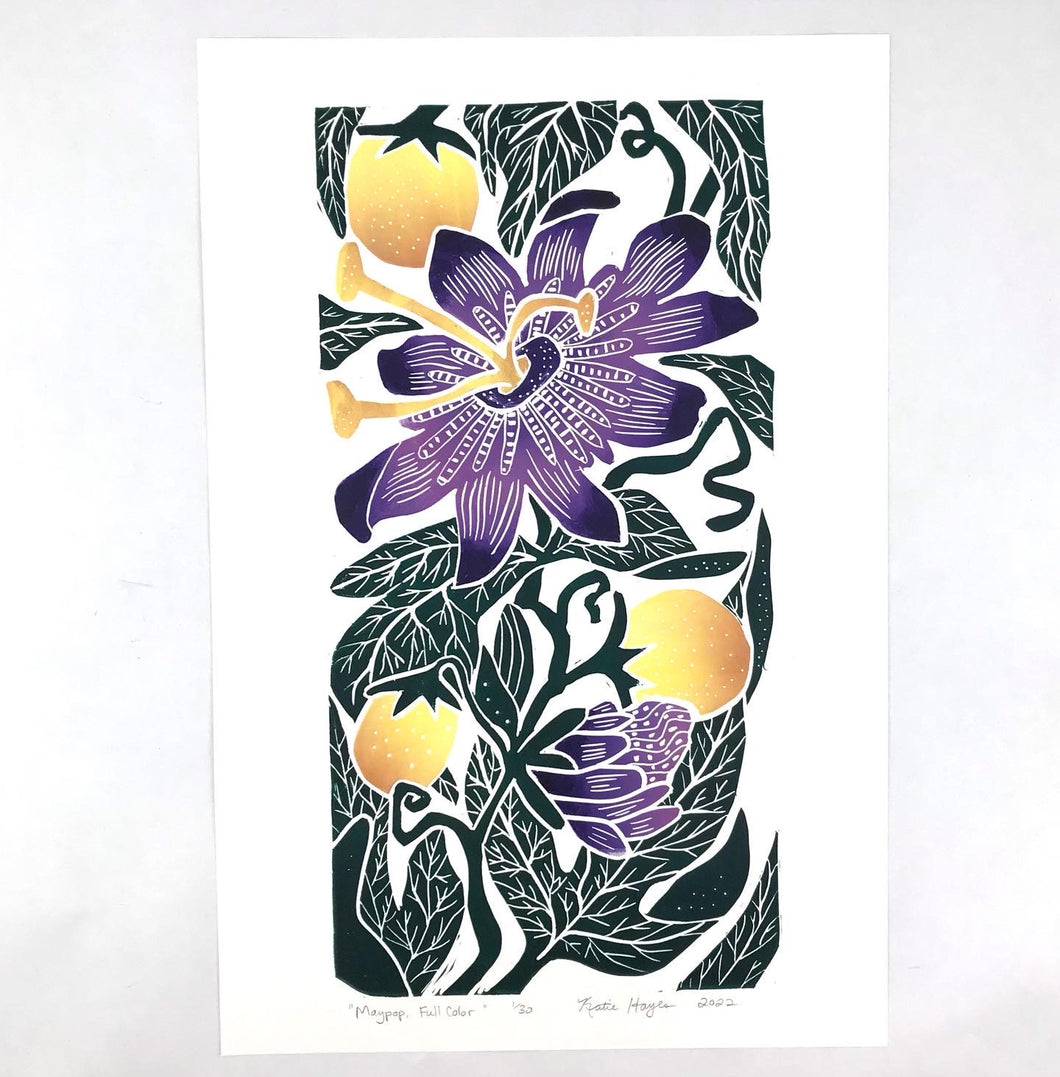This artwork by Christy Hagen, titled "Meg Pipe Full Color 20 Schritt," created in 2022, is a vertically rectangular (portrait mode) piece that features a detailed botanical illustration set against a white background with gray borders. At the center and bottom of the composition are two purple flowers, one open and one closed, each held up by a black stem. The open flower showcases three prominent, long yellow-orange stamens emerging from its center. Surrounding the central purple flower, there are three peach-colored fruits. Additionally, the artwork includes green leaves with distinct white veins, some of which support yellowish buds or bulbs. The text "Meg, Meg, Pipe, Full Color, 20, Schritt" is located at the bottom of the image.